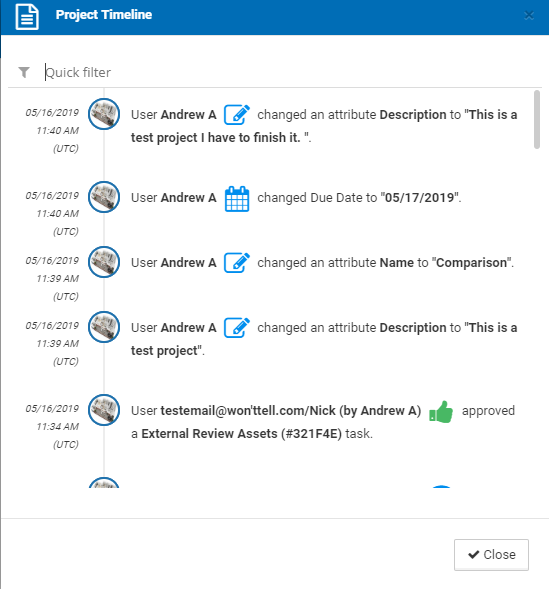A detailed project timeline of user activities is displayed, capturing updates made by User Andrew A on May 16, 2019. The timeline spans from 11:34 AM to 11:40 AM, showcasing five distinct visual scenes:

1. **11:34 AM** - User Andrew A (bolded) changed the due date of a task.
2. **11:36 AM** - User Andrew A modified the name associated with a person.
3. **11:37 AM** - User Andrew A updated the description of a task or item.
4. **11:39 AM** - User Andrew A approved a specific change.
5. **11:40 AM** - A final scene summarizing the updates, illustrated with a circle containing an image on the right side, while detailed descriptions of each action are presented on the left.

A quote filter tab is also visible, providing additional context or filtering options for the timeline.